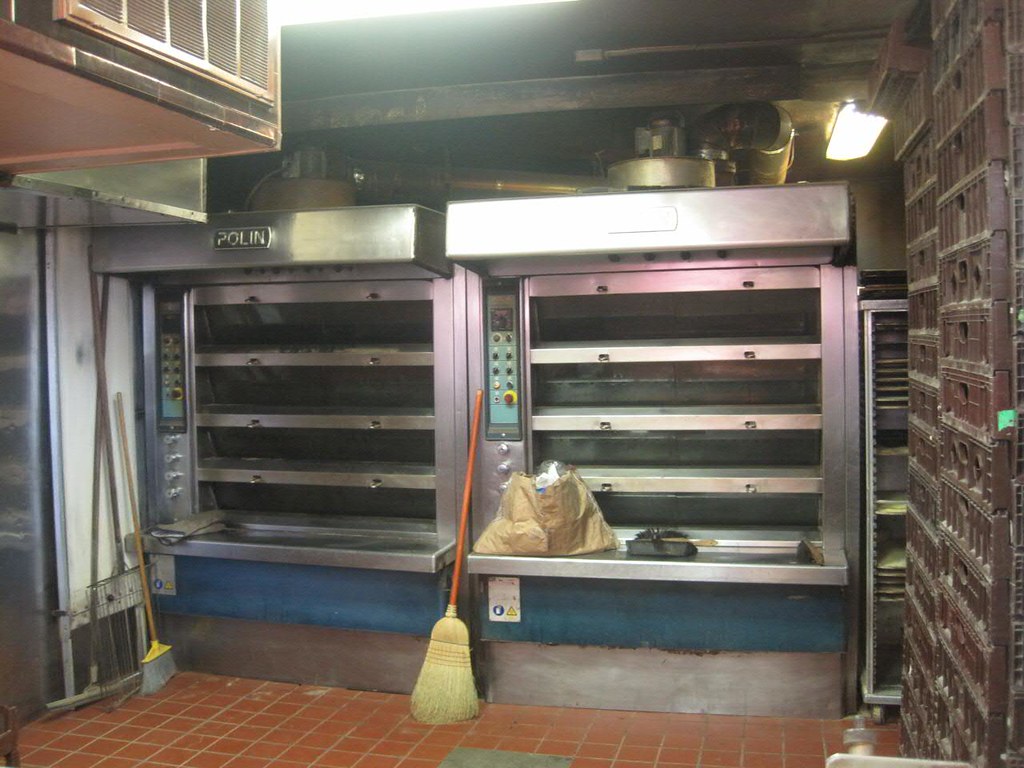The photograph depicts the interior of a restaurant kitchen with notable features and equipment. The floor is tiled in a burnt orange color, contributing to the industrial ambiance. Three brooms are visible, with one propped against a metal wall while the other two are centralized within the kitchen area. Dominating the scene are two large double ovens, each with four compartments, characterized by a mix of silver, blue, and metallic colors. The ovens feature control panels with green, yellow, and white knobs, and beneath them is additional metal piping, possibly part of the ventilation system.

On the left side of the kitchen, a brick wall rises past a metal wall, complemented by a white ceiling. The ceiling houses an old air conditioning unit and adequate lighting. On top of the ovens, a ventilation system is clearly visible. There are various pieces of equipment scattered, including a grocery bag and a dustpan. Additionally, on the right side, there are brown crates stacked up to the ceiling, adding to the clutter typical of a busy kitchen. The wall also includes a silver door and a prominent sign with the lettering "P-O-L-I-N."